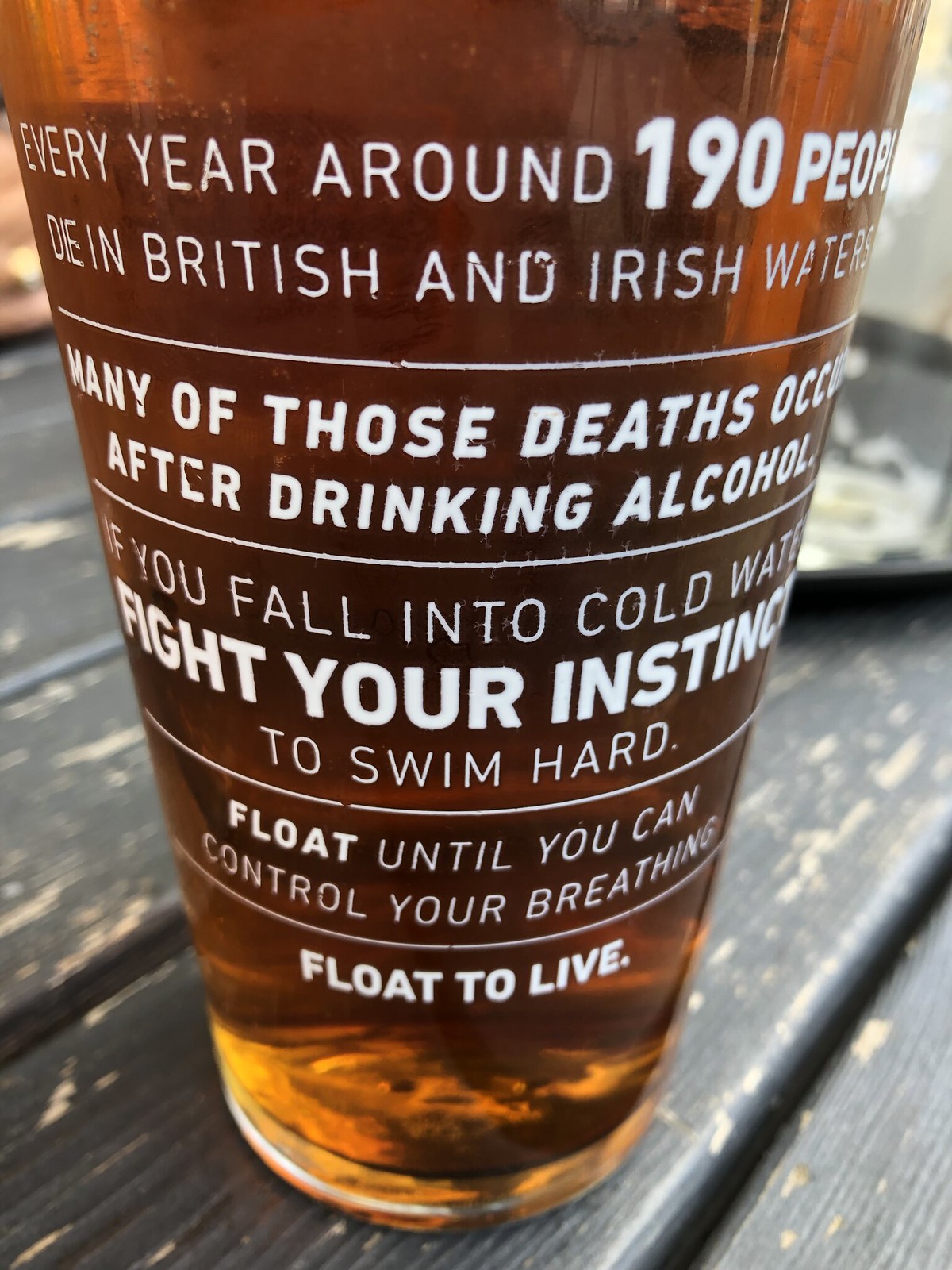The image features an up-close shot of a beer glass filled with an amber-colored liquid, possibly beer, sitting on a weathered wooden tabletop that has been painted black but now shows signs of chipping. There is a blurry plate mostly behind the glass on the right-hand side, barely in focus. The main focus of the image is the white text printed on the glass, which reads: "Every year around 190 people die in British and Irish waters. Many of those deaths occur after drinking alcohol. If you fall into cold water, fight your instincts to swim hard. Float until you can control your breathing. Float to live." The text is presented in various sizes and includes some bold fonts, making the critical message stand out. Light filters through the amber liquid, adding a warm glow to the scene.